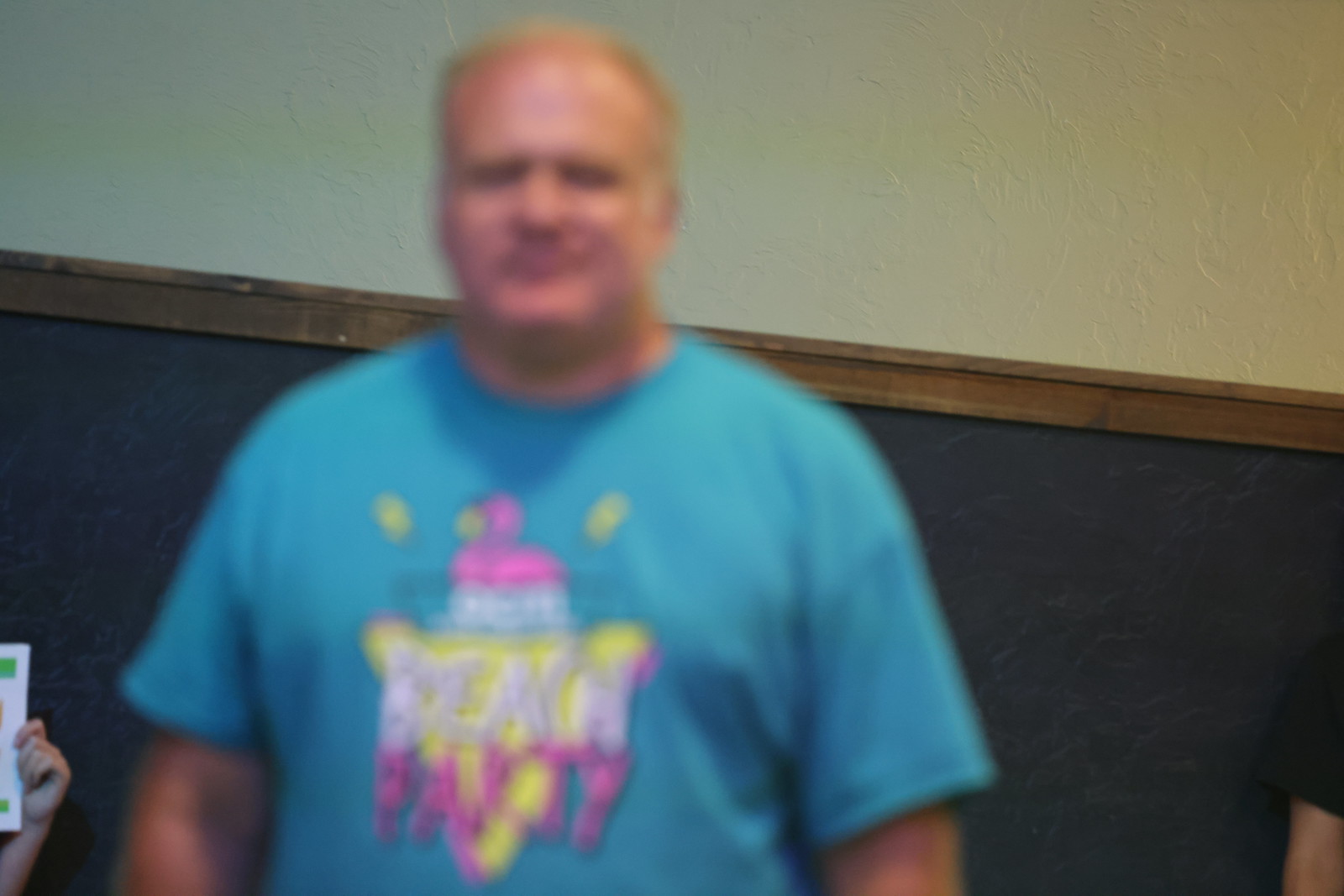In this slightly blurry photograph, a light gray wall serves as the backdrop, accentuated by a dark gray chalkboard framed in brown wood. Standing in front of the chalkboard is a middle-aged man with short blonde hair, smiling warmly. He is dressed in a light blue short-sleeved t-shirt featuring a colorful design with pink, white, and yellow elements, including a triangle shape with a white top and some text in pink and white. To the side, a child's hands are visible, holding up a piece of white paper adorned with green markings. Additionally, an arm clad in a black shirt from another young person can be seen, contributing to the lively and engaging atmosphere of the scene.